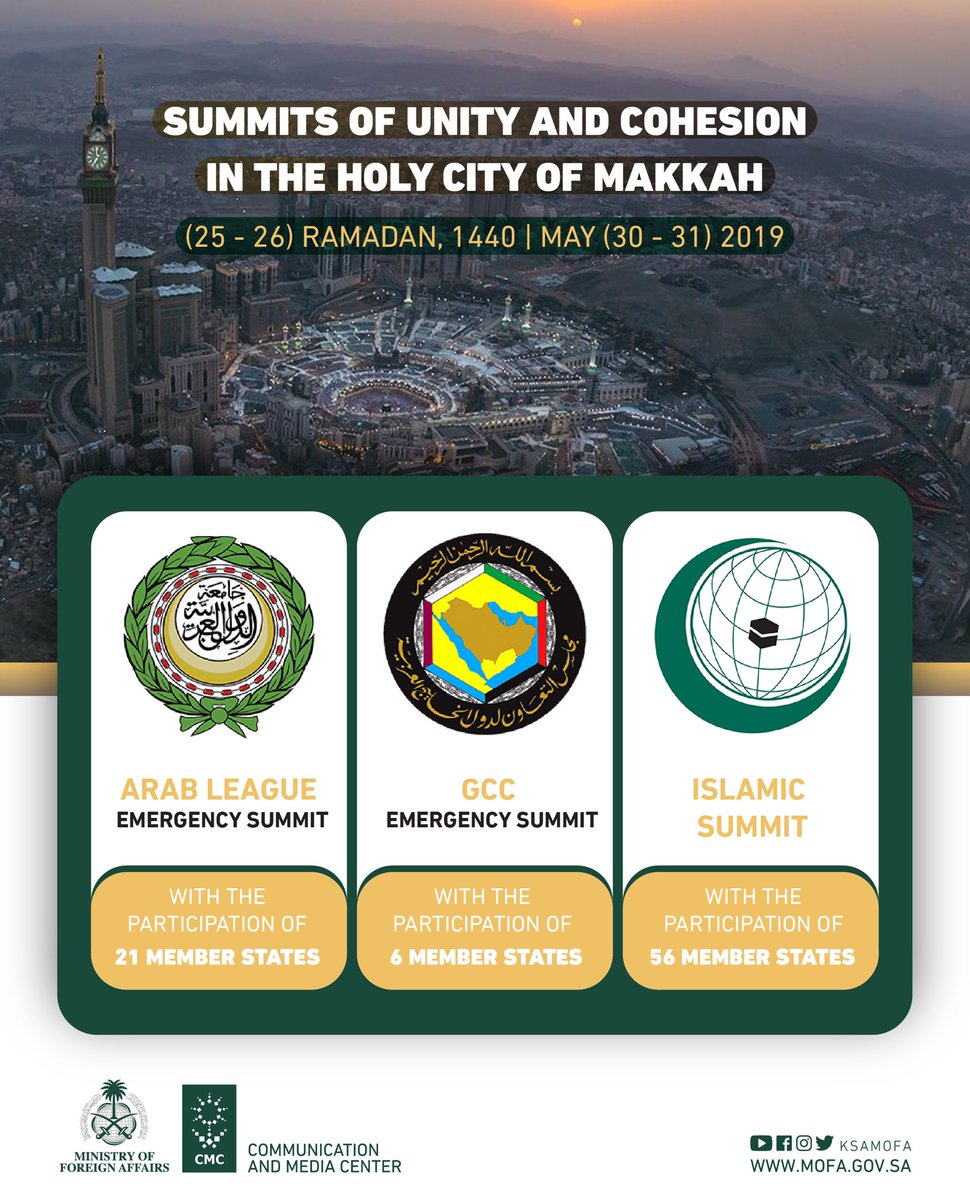A promotional image depicts a significant event taking place in a large city, likely Mecca, based on the context. The background, occupying about half of the image, features a photograph of a grand cityscape at sunset. Prominent in the photo is a gated community labeled "Summits of Unity and Cohesion in the Holy City of Mecca," with the dates "25 through 26 Ramadan, 1440 (May 30th through 31st, 2019)" included in parentheses underneath. On the left side of the backdrop, a tall clock spire rises against the skyline filled with towering buildings, while the right side shows expanses of green space, suggesting residential communities.

In the foreground, three vertical rectangular banners provide additional information about the events. The banner on the left announces the "Arab League Emergency Summit" with participation from 21 member states. The center banner details the "GCC Emergency Summit" with six member states taking part. The right banner highlights the "Islamic Summit," noting participation from 56 member states.